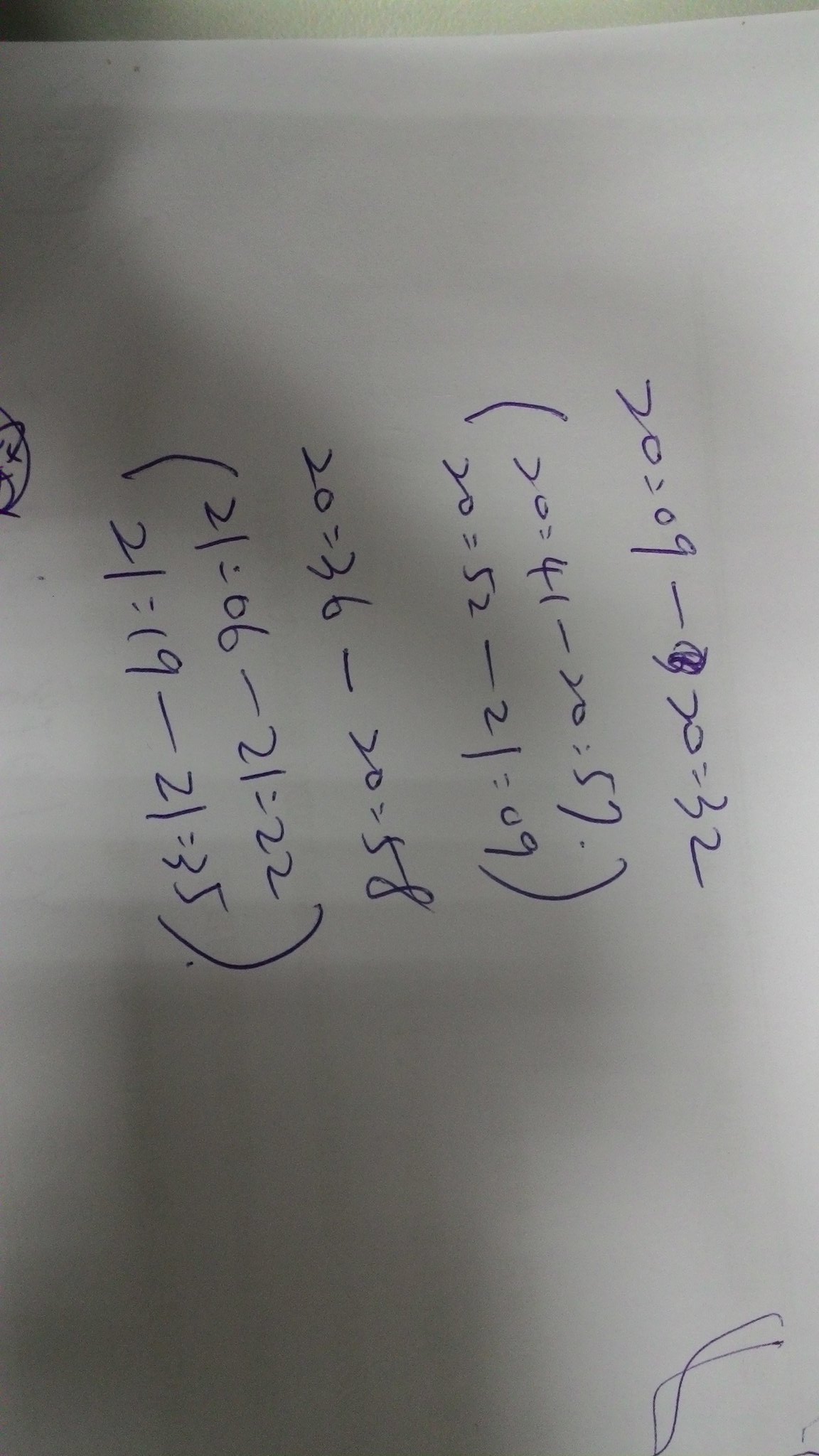This color photograph captures a piece of white paper with gray shadows, showcasing handwritten mathematical formulas in blue ballpoint pen ink. The handwriting, although slightly difficult to read, features complex equations and numerical values organized into six rows. Despite the portrait orientation of the image, the writing itself appears sideways, adding to the challenge of deciphering the content. Each line follows a structured pattern involving numbers, subtraction, and parentheses. The first line reads: "20 = 09 - 20 = 32 (20 = 41 - 20 = 57)". Subsequent lines display similar arithmetic sequences: "20 = 52 - 21 = 09", followed by "20 = 36 - 20 = 58 (21 = 06 - 21 = 22)". The final line states: "21 = 19 - 21 = 35". This photograph provides an intricate glimpse into handwritten mathematical problem-solving.